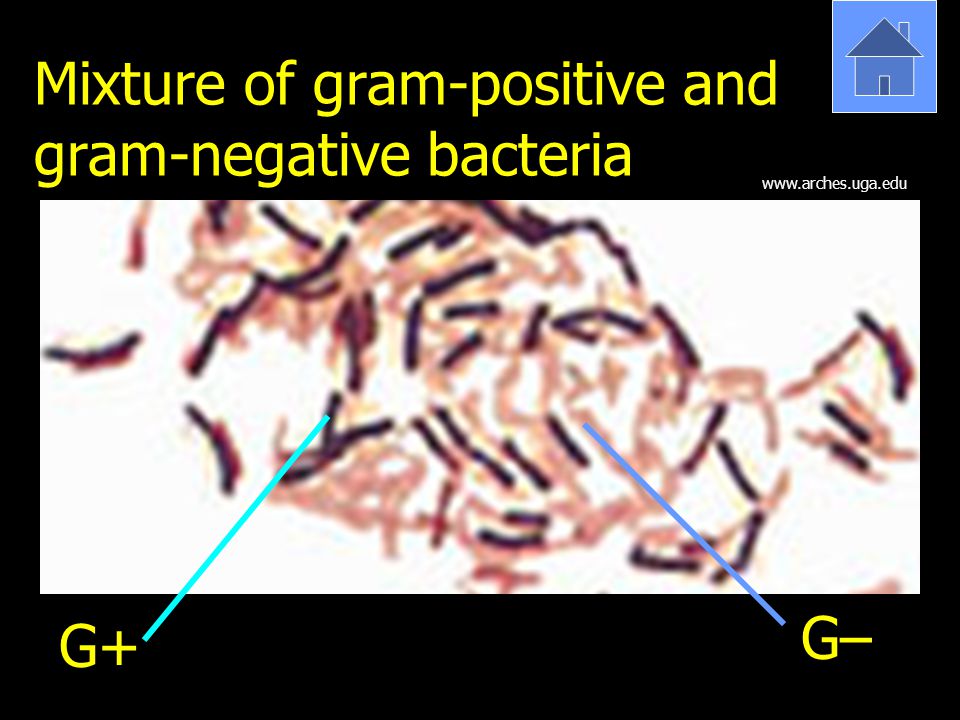The image features a rectangular layout akin to a business card, predominantly bordered in black. The card’s top right corner showcases a simplistic clipart logo of a house with a triangle roof set against a dark blue background. Centered on this card and prominently displayed in bright gold lettering is the title, "Mixture of Gram-Positive and Gram-Negative Bacteria". Beneath this title, there is a detailed depiction of bacteria as seen through a microscope, featuring small lines in shades of pink, salmon, peach, dark purple, and black. 

The lighter pink and peach strands represent Gram-negative bacteria, labeled with a blue line pointing to the right along with a "G-". Conversely, the darker purple strands signify Gram-positive bacteria, marked by another blue line on the left leading to a "G+". The background behind the microscopic imagery remains black, creating a distinct contrast with the colorful lines. Below the top right house logo, very small white text displays the website "www.arches.uga.edu". The composition suggests an educational context, possibly a slide from a science lecture or a presentation, demonstrating the visual differences between Gram-positive and Gram-negative bacteria.